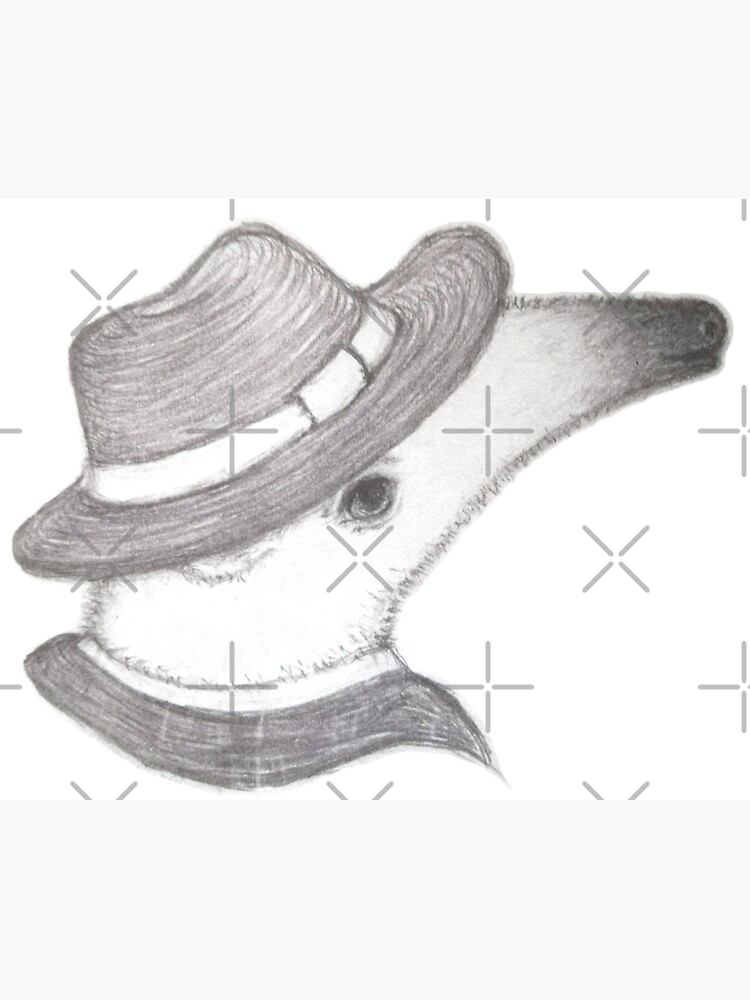This is a whimsical, pencil-drawn illustration on a white background, overlaid with transparent crosshairs, suggesting it is from a stock photo website. The image depicts an anthropomorphized anteater with distinctive features. The anteater has a white head and a long, darker-colored nose that integrates with its mouth, exhibiting a single visible eye positioned on the side of its head. It's adorned in a vintage ensemble: a darkly shaded fedora hat with a white band, giving it a textured, fuzzy appearance, and a suit jacket featuring a white collar and dark shoulders, evoking an old-time, possibly 1950s, aesthetic. The drawing’s playful nature and detailed attire suggest a character reminiscent of a retro gangster or a businessman from the mid-20th century.